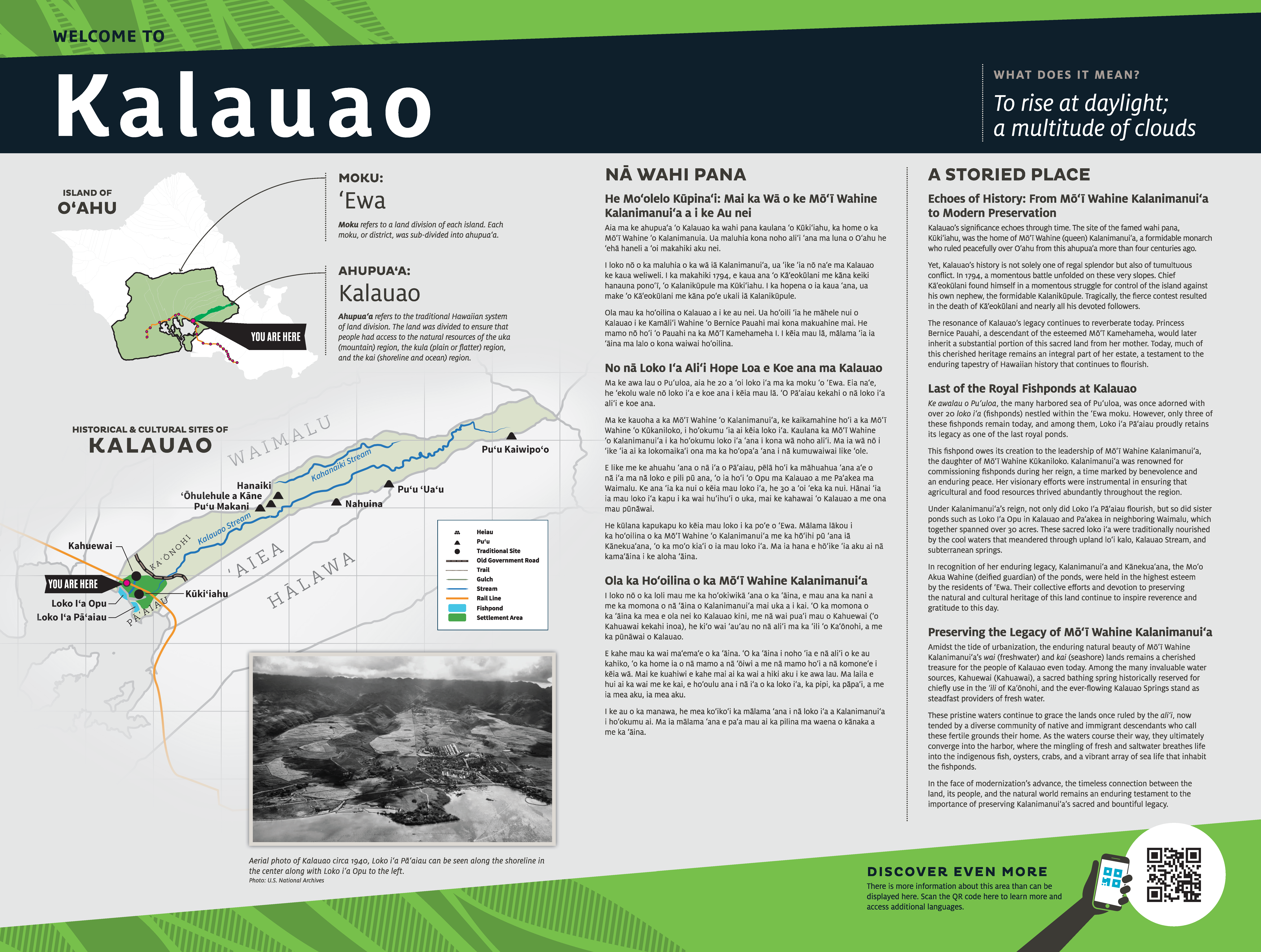This image appears to be an advertisement or informational brochure for Kalawao, a location on the island of O'ahu in Hawaii. The top of the image prominently features the greeting "Welcome to Kalawao" in large white letters. To the right of this title, the text explains the meaning of Kalawao as "to rise at daylight, a multitude of clouds."

Beneath this main title, there is a map of O'ahu showing the specific location of Kalawao, supplemented by another, more detailed map below that includes site illustrations and markers indicating "You Are Here." The detailed map highlights important historical and cultural sites, and there is additional information about the rivers in the area.

To the right of these maps, a section is divided into two columns; the left column appears to be in the native Hawaiian language and the right in English, titled "Nawahipana" and "A Storied Place," respectively. The English text expands on the history of Kalawao, discussing significant elements such as the last of the royal fishponds and the ongoing efforts to preserve the island's cultural legacy.

The overall color scheme of the image is green and gray, enhancing the natural and historical themes presented. The layout and detailed descriptions suggest that the image is designed to be both informative and easily understandable, serving as an educational guide to the area.